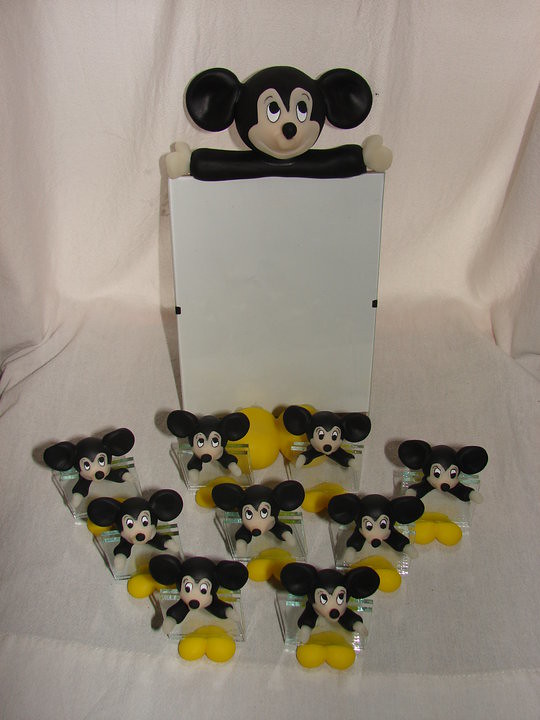In this detailed photograph, set against a backdrop mimicking a white curtain or blanket, a display of mouse toys is featured prominently. The focal point is an oversized mock-Mickey Mouse figure, with black ears positioned more towards the sides of its head. Its tan face showcases distinct eyes, a nose, and a mouth. This main figure extends its black arms horizontally, ending in beige hands. It appears to lean against a large white rectangular object, possibly a dry erase board, partially obscured by the draped sheet beneath it.

Beneath this primary figure, nine smaller mouse toys, resembling vintage or knockoff Mickey Mouses, are meticulously arranged in a triangle formation. These miniature figures bear black ears, tan faces, and black arms. Unlike the large figure, these smaller toys rest on plastic yellow feet and seem to incorporate small glass squares beneath their arms. The entire display is positioned on what appears to be a hard surface, covered by the same white material, with green bars faintly visible behind the toys, adding to the structured setup of the scene.